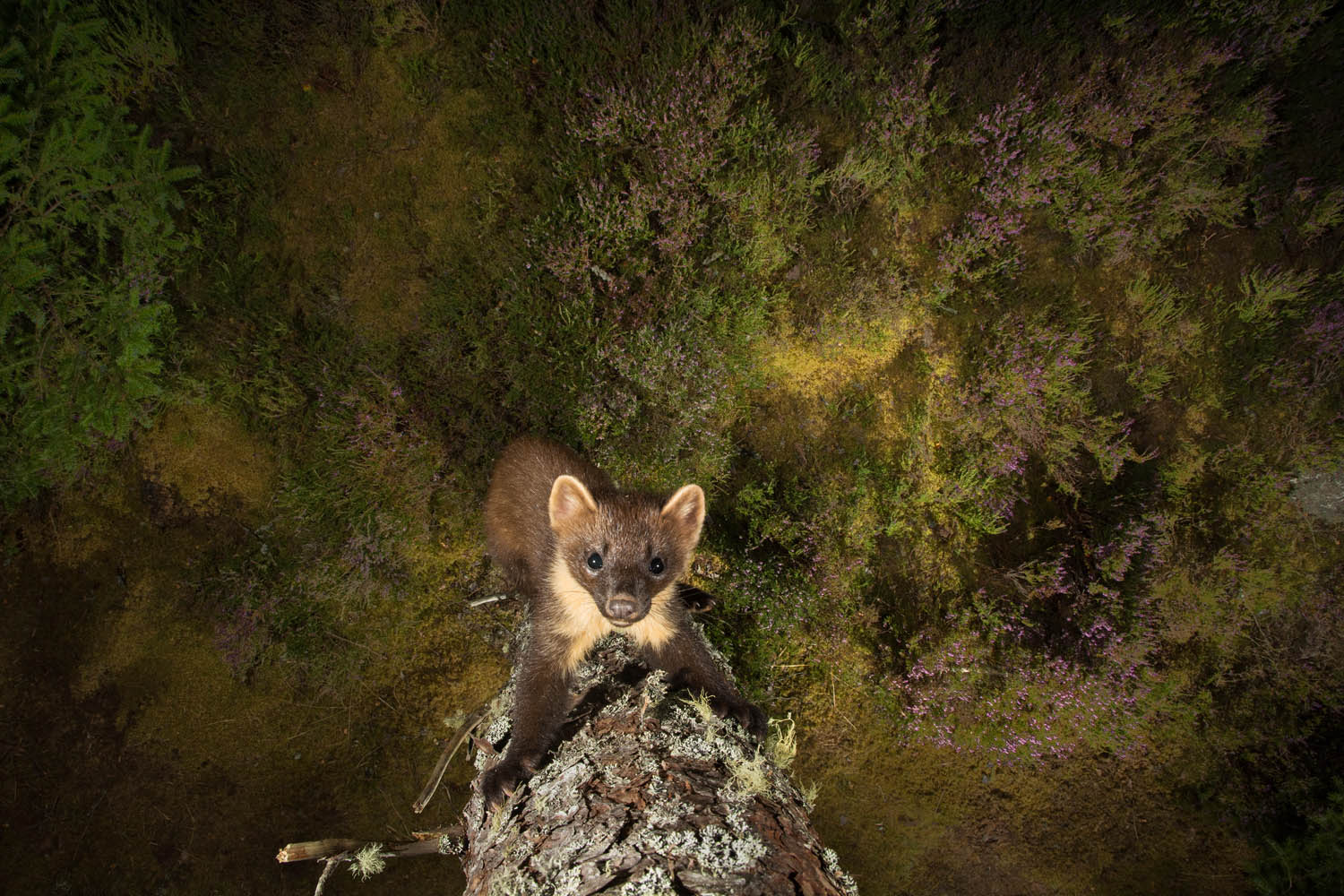This image captures a nocturnal scene, illuminated by flash, revealing a small, seemingly bear-like animal climbing a pine tree. The creature, perhaps resembling a panda, raccoon, or Tasmanian devil, has a dark brown body with lighter, tan fur around its pointy ears and neck. It sports a brown snout and its inquisitive face is turned towards the camera. The texture of the tree's trunk, which appears relatively thin and laden with grooves, is clearly visible. The background showcases a diverse forest floor speckled with various trees, shrubs, and bushes in shades of brown, green, and yellow, contributing to the dense woodland setting. The tree branch or log, bearing a whitish-gray, ash-like hue, further frames this enigmatic forest inhabitant as it clambers upwards in the serene night.